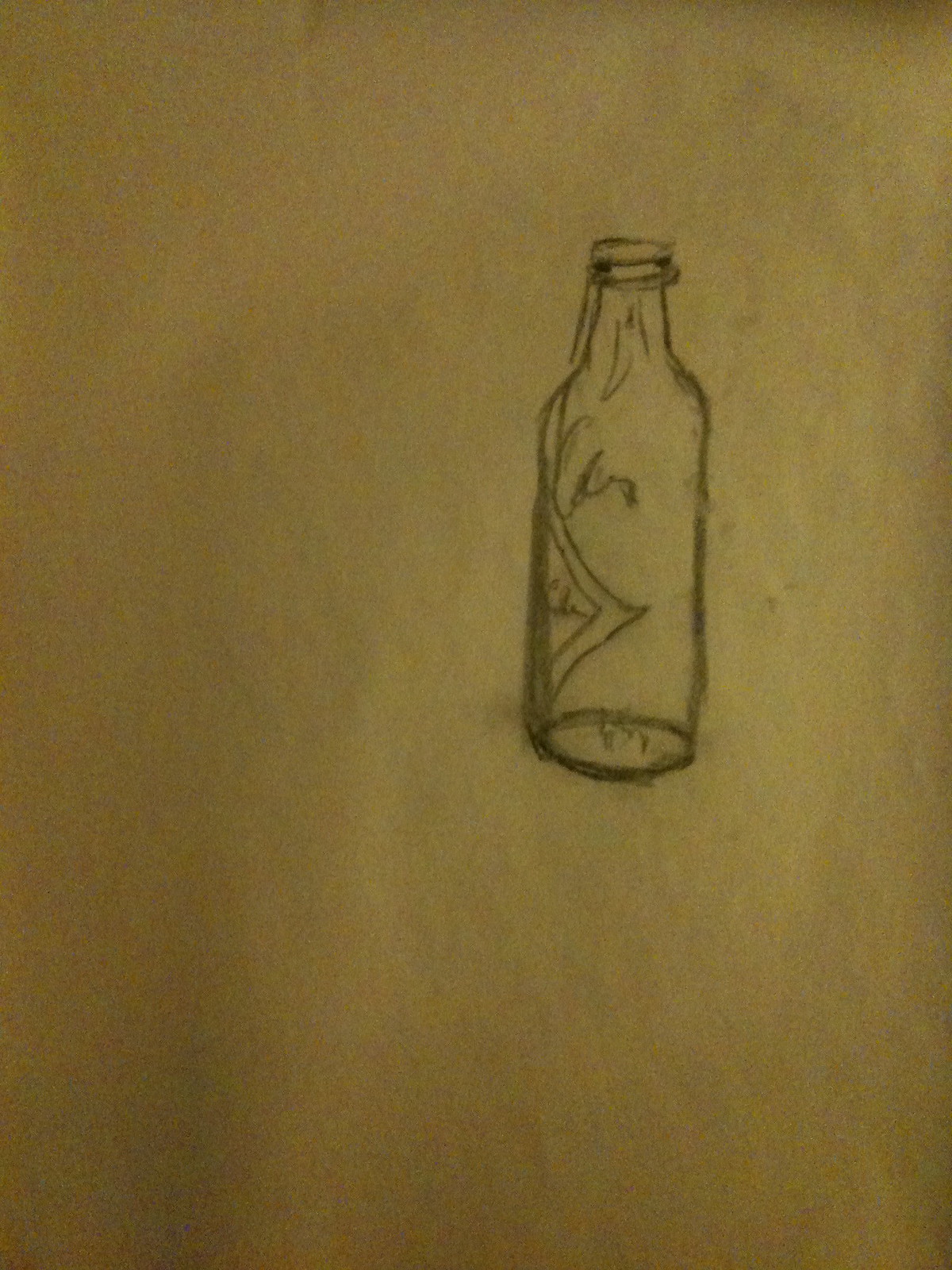The image depicts a hand-drawn pencil sketch of a clear, empty glass bottle seen slightly off-center towards the right against a yellow, aged-looking paper background. The bottle is well-proportioned, with a neck that aligns perfectly with the body's straight shape. It features a rounded base and an open neck. The drawing appears moderately refined, indicating some artistic skill but still retains a beginner's touch, noticeable in areas where lines were redrawn, particularly on the left side of the bottle. A partial diamond-shaped pattern, possibly intended as a label, is visible on the left side of the bottle. Despite the evident effort in the sketch, there is some scribbled text and a double-lined "V" shape on the underside. There is no indication of liquid inside the bottle. The paper’s background, which looks tan and brown due to shading or possibly due to the dark photograph, contributes to the overall aged appearance of the artwork.